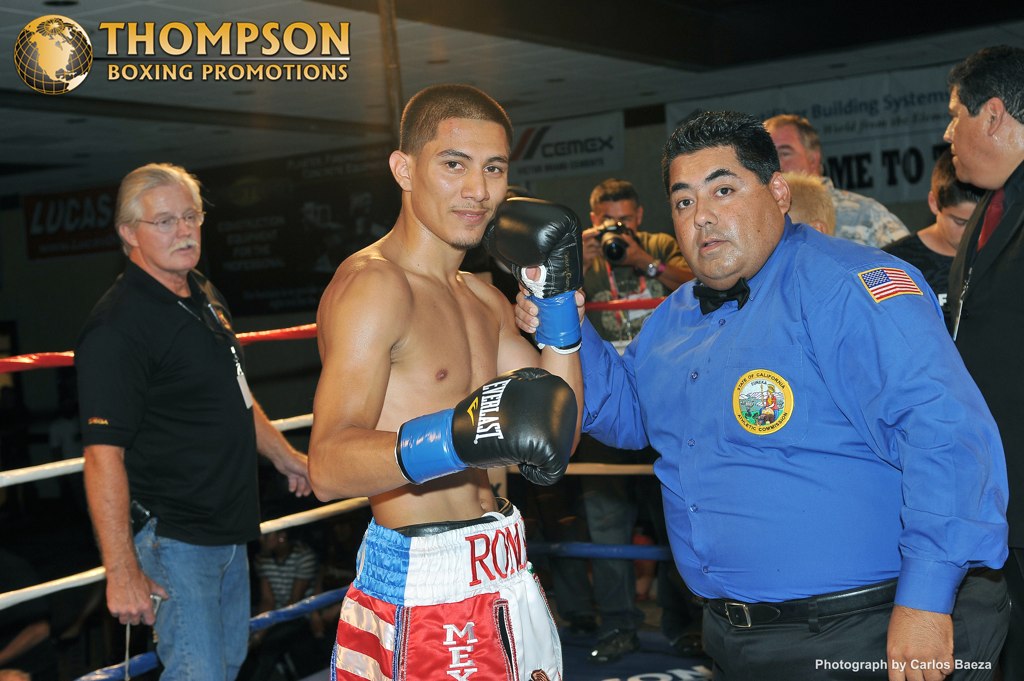This detailed color photograph, taken inside a gymnasium boxing ring, captures a young, shirtless boxer in the center. He has short black hair, slight stubble, and is wearing black boxing gloves along with red, white, and blue trunks. The boxer holds his gloves in a formal boxing stance, his left glove touching his cheek, and smiles slightly into the camera. Standing next to him on the right is a large man, possibly a judge or security officer, dressed in a long-sleeved blue button-down shirt adorned with an American flag patch on the right shoulder and a circular State of California Athletic Commission patch on his chest. This man, with black hair and a slightly chubby build, grasps the boxer’s left wrist, signifying the declaration of the fight's winner. In the background, several photographers are seen capturing the moment, including a prominent figure between the two main subjects holding a small black camera. An older man with a big white mustache, wearing a black shirt and blue jeans, is also visible to the left. The top left corner of the image features the logo "Thompson Boxing Promotions" overlaid on a globe focused on North America. In the bottom right, the photograph is credited to Carlos Bezos.